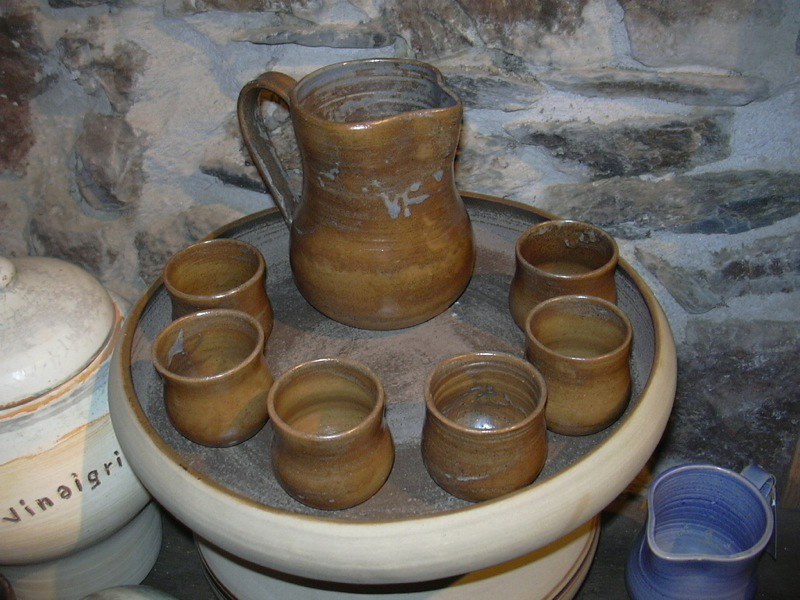This image showcases a collection of handcrafted pottery pieces arranged against a rustic backdrop of a grey, brownish stone wall with visible cement or concrete in between the stones. Nestled on a small white table, there is an assortment of six light brown cups, each adorned with unique brown swirls, giving them a traditional, hand-made appearance unlike factory-produced items. Centrally placed among these cups is a larger brown pitcher with a handle, suggestive of its use for pouring. Indicating its artisanal nature, the pitcher features the letters "V-W" in a grey tone.

To the left side of the image, there is a distinctive light brown pot with a white lid, bearing the hand-written inscription "V-I-N-A-I-G-R-I" in dark brown letters, further emphasizing the manually crafted feel. Adding contrast to the earthy tones, a striking blue and white pitcher is positioned at the bottom right corner. This vivid blue pitcher stands out against the otherwise warm palette of browns and whites. The overall setting, with its wooden wall background and the mix of functional pottery, evokes a sense of traditional craftsmanship and historical lifestyle.